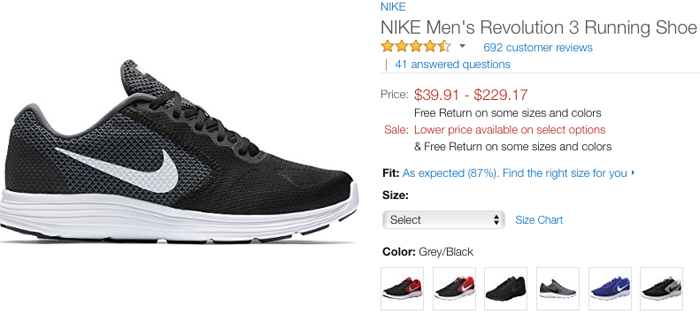Close-up of a Nike shoe, specifically the right foot, positioned with the heel on the left and the toe on the right. The thick sole is completely white, contrasting against the black bottom. A prominent white Nike swoosh is clearly visible. The upper part of the shoe is predominantly black, with a mid-section featuring a blend of charcoal gray and black hues, adorned with an additional Nike swoosh.

The laces are neatly crisscrossed, though the bow is not visible. The shoe is displayed on its own, not being worn. The design is labeled as the Nike Men's Revolution 3 Running Shoe. Accompanying information indicates that it has received 602 reviews, boasting an average rating of 4.5 stars. Pricing for this shoe ranges from $39.91 to $229.17, with free returns available for certain sizes and colors. The lower price is applicable only to selected options, and 87% of reviewers report that the shoe fits as expected. Additionally, the shoe is available in a variety of colors, with six alternative options displayed at the bottom right corner of the image.